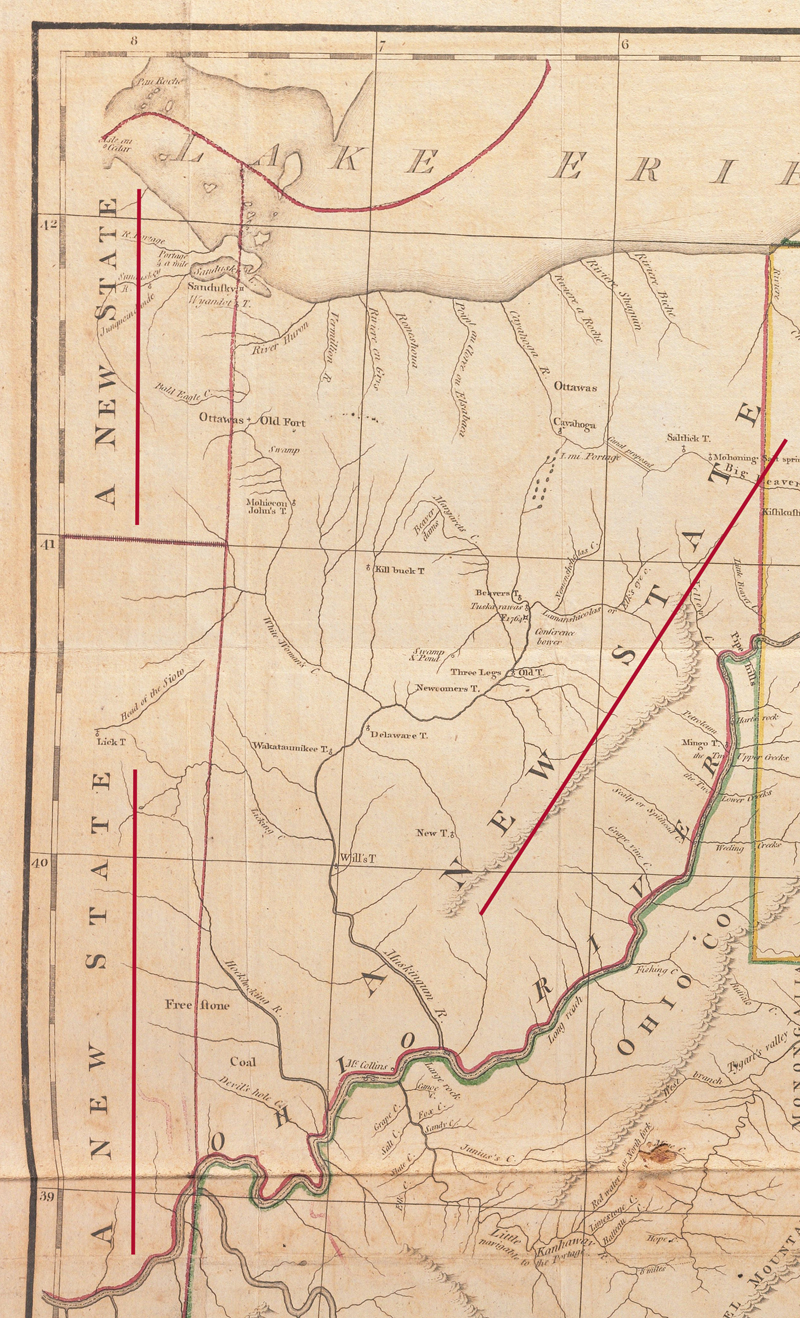The image appears to be a photograph of an antique map, likely extracted from an atlas. The map is centered around Ohio and prominently features the Ohio River and possibly Lake Erie at the top, although the latter is partly cut off. The design is monochromatic with a beige background and black borders, supplemented by red lines marking state boundaries and various regions. The map also highlights numerous smaller towns and geographical features such as rivers, roads, and mountains. The text "new state" can be seen repeatedly on the map. However, the map is incomplete—nearly half of it is cut off, obscuring much of the detail, including anything to the right of "Ohio Co." The map seemingly indicates areas up to the border of Canada, evidenced by a partial reference to Ottawa, though this is not distinctly clear. The map is enhanced with visible fold lines, suggesting its age and usage over time.